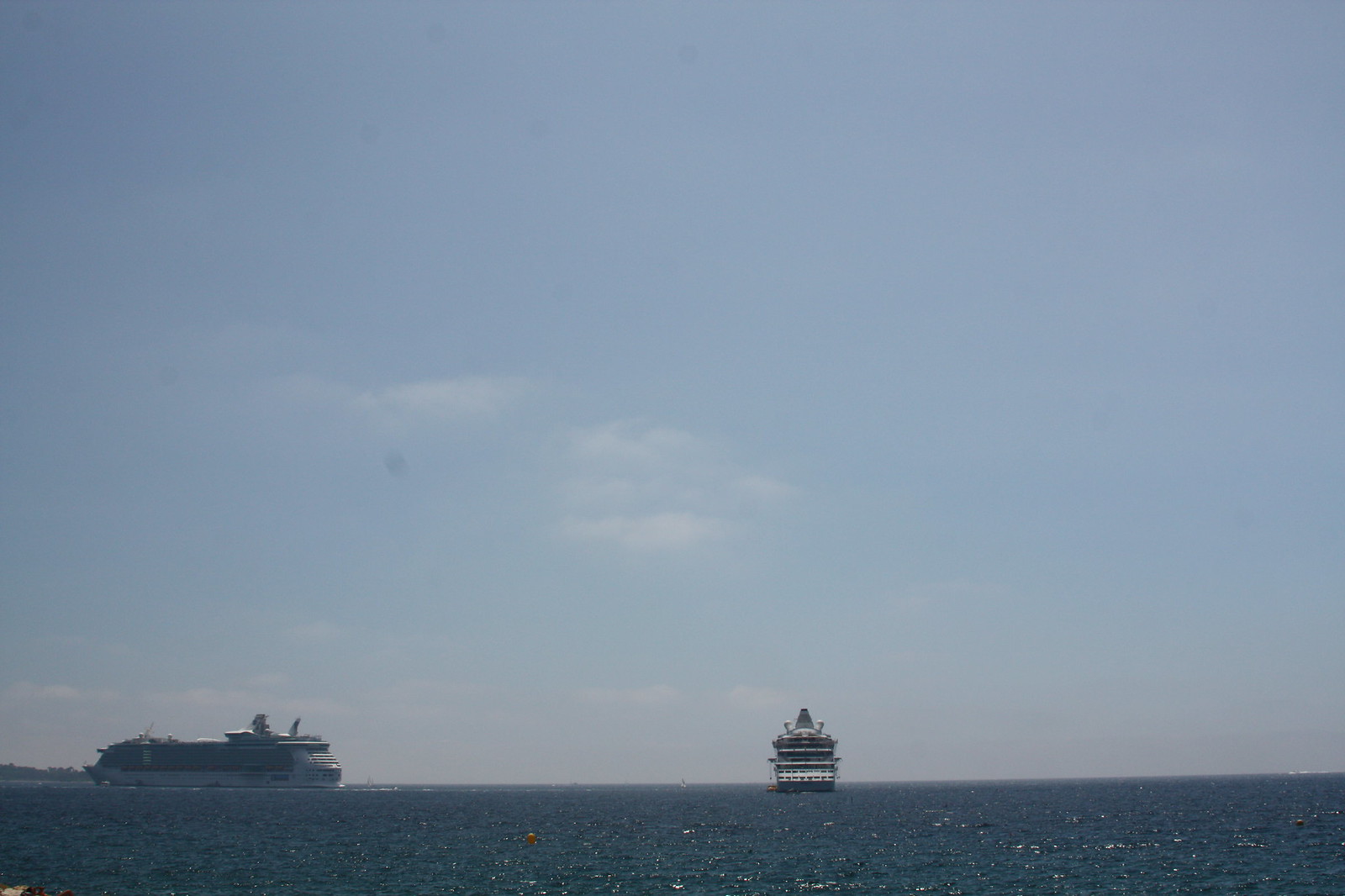This photograph captures two large ships on a calm ocean under a vast, predominantly blue sky. The sky, occupying around 80% of the image, features a few wispy clouds and a slight pinkish hue near the horizon. The water below is a deep blue with a gentle chop, filling the remaining 20% of the frame. On the horizon, there is a faint glimpse of land toward the far left.

The two ships, possibly cruise or passenger ferries, dominate the central focus. The ship on the left is viewed horizontally, giving a clear profile that reveals its large white structure and multiple levels, indicative of a cruise ship. The ship on the right appears to be positioned either directly facing or moving away from the camera, making its full scale harder to discern. This ship too exhibits white and black coloring, possibly with white railings.

Overall, the composition is serene and balanced, effectively utilizing the interplay of sky and sea to frame the two distant vessels.